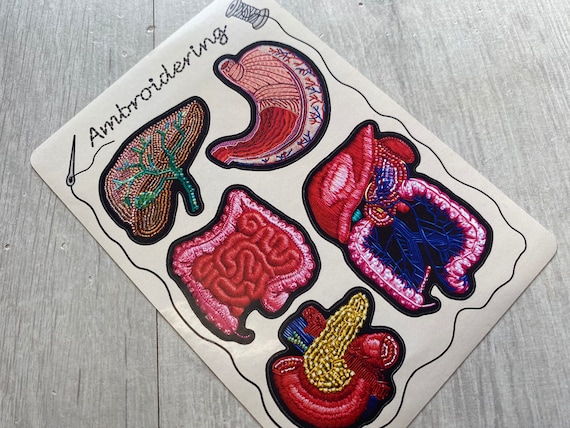The image depicts a white piece of paper placed on a whitewashed wooden floor. The paper prominently displays the word "EMBROIDERING" in a stitched-like font at the top. Surrounding the paper is a black and white spool of thread, which unwinds and wraps around the edges of the paper, eventually threading through a needle positioned near the title.

On the paper itself, there are five embroidered images of human organs. In the top left corner, an embroidered brain is visible, featuring green veins and intricate details. Opposite the brain, in the top right corner, is an embroidered heart. Below the embroidered brain, to the left, is an intestinal system rendered in red with surrounding pink body tissue, capturing both the large and small intestines vividly. Directly beneath this, there is an embroidered depiction of heart valves. To the right of this image, and completing the collection, is another embroidered organ that appears to be a part of the digestive system. Each of these colorful, detailed embroideries appears on the paper as if they could be iron-on patches or stickers. The overall image is artistically laid out, resembling a carefully assembled plaque of embroidered anatomical art.